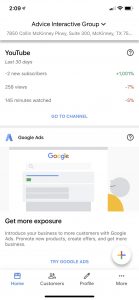Screenshot of an analytics page for Google products. At the top, it is titled "Advice Interactive Group" with other text beneath it appearing blurry, likely an address. Below a grey line divider, the page features the bold black text "YouTube" followed by the phrase "last 30 days." The analytics indicate "two new subscribers" in blurry text. Below this, there is a blue link labeled "Go to channel" and another grey line divider. The next section is titled "Google Ads" and showcases a sample webpage with the Google logo at the top. The page contains several grey rectangles and the text "Get more exposure." At the bottom of this section, there are three lines of text with a blue link: "Try Google Ads." Additionally, there is a circle-shaped plus button located in the bottom right corner.